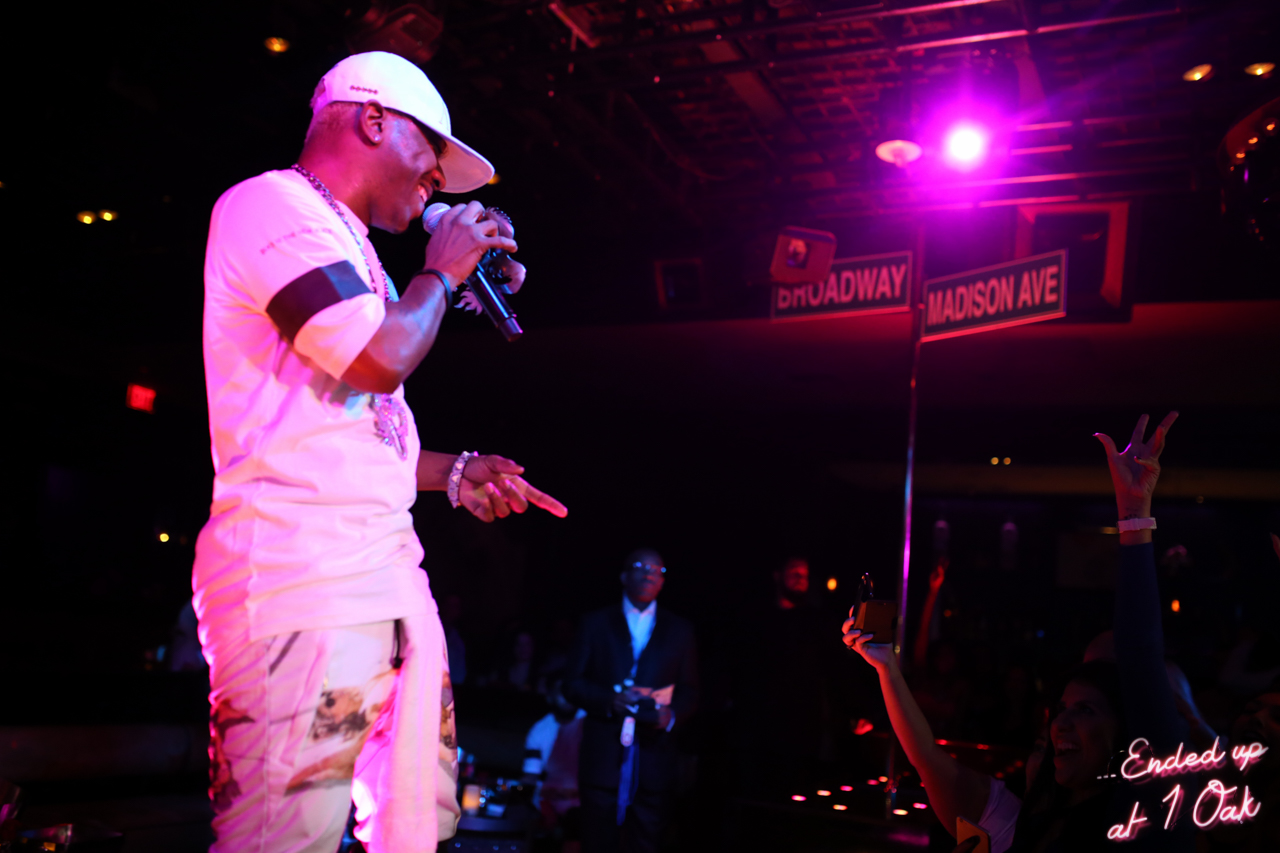The image captures a vibrant nightclub or concert scene, suggesting a performance environment. Emerging prominently from the background crowd, a man adorned in a white ensemble stands out. He wears a short-sleeved shirt with a black armband around his right bicep, white pants, and a white baseball cap. In his right hand, he grips a microphone, seemingly in mid-performance or addressing the audience, while his left hand points outward. His wrist bears a wristband that adds to his distinct look. The upper portion of the image is illuminated by a pink spotlight, which casts a glow on road signs that read "Broadway" and "Madison Avenue" in red on black. These street signs create an intriguing backdrop that juxtaposes the nightclub vibe. The lower right corner of the image features a neon script font that reads "Ended Up at One Oak," indicating the well-known club, likely located in the Mirage, Las Vegas. Silhouetted figures in the background enhance the lively and immersive atmosphere of the venue.